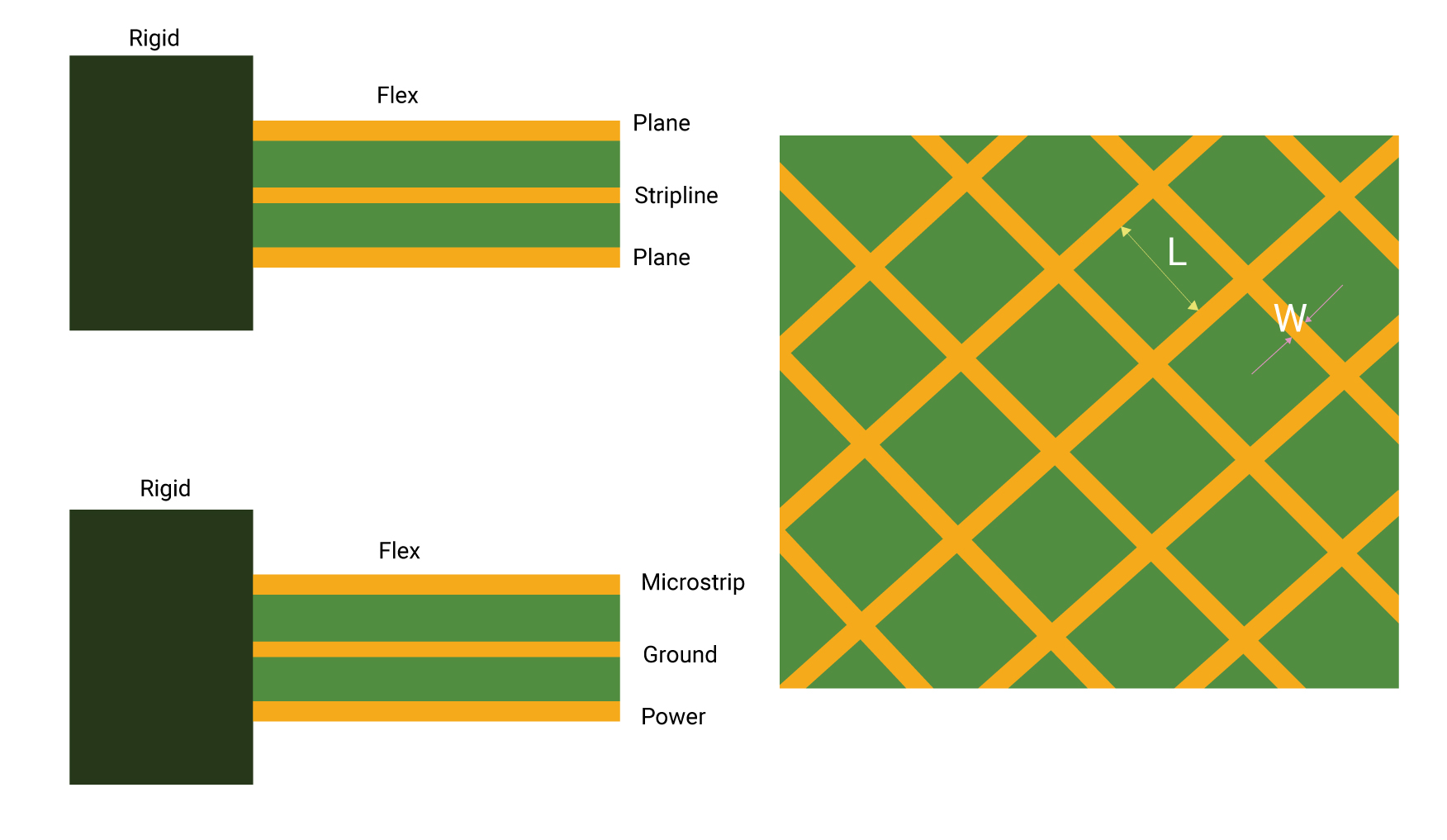The image features a detailed, checkered pattern dominated by green and yellow hues. On the right side, there is a large square with a yellow cross-hatch pattern and smaller green squares within it. Overlaid near the top-right corner of this square, there's a white "L" marked by a pale yellow line running its length, and a "W" accompanied by two purplish lines pointing inward. Adjacent to this large square, continuing to the left, are two identical patterns each containing a dark green vertical rectangle connected to a thinner, horizontally striped lighter green and yellow rectangle. The top of the dark green rectangle is labeled "rigid," and the horizontal rectangle is labeled with texts like "plain," "strip line," and "plain" again. Below this, a similar pattern repeats but is labeled "microstrip," "ground," and "power." The meticulous arrangement and the distinct labeling present a structured and informative illustration that seems to blend elements of plaid design with textual annotations.